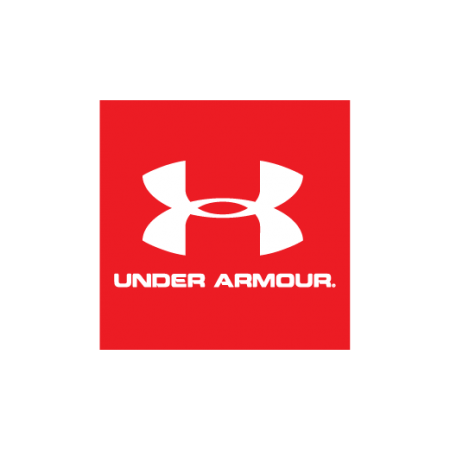The image is a square with a solid bright red background. Centrally positioned is the iconic Under Armour logo in white. This logo consists of two stylized semicircles: the top one starts upward, dips down in the middle, and ascends again at the ends, which are thicker than the middle section. The lower semicircle starts downward, curves up to intersect with the top semicircle, then descends on the right, also with thicker ends. The intersection of these semicircles creates an oval shape, revealing the bright red background through the center. Below the logo, the brand name "UNDER ARMOUR" is prominently displayed in all capital letters with a white font. Notably, "ARMOUR" is spelled with a "U" as in British English. There appears to be a period or a small symbol following the brand name. The entire composition is centered, maintaining equal distance from all sides, creating a balanced and visually appealing presentation.